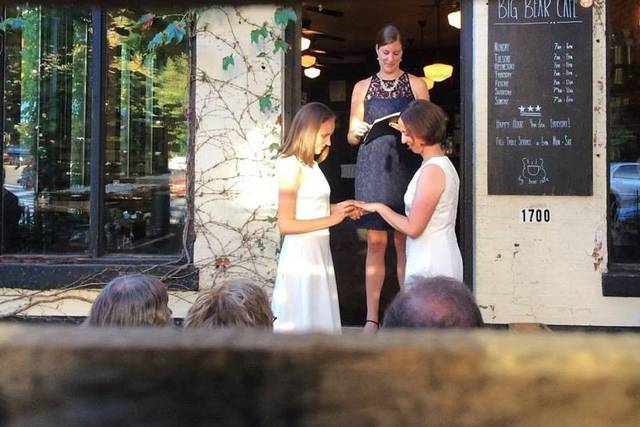The image captures a realistic and intimate wedding ceremony, likely at a local establishment named Big Bear Cafe, located at 1700, as indicated by the signage. The photograph is horizontally oriented and appears to be taken from the perspective of someone peering over a wooden fence. Two Caucasian women in their 20s or 30s are at the center of the ceremony, both elegantly dressed in white gowns, holding hands, and seemingly exchanging rings. Behind them, a third woman in a dark dress, possibly black or dark blue, is presiding over the ceremony, holding and reading from a book—potentially the vows. The cafe's setting features beige stucco-style walls adorned with vines, large windows reflecting the surroundings, and a menu or schedule posted beside the open doorway where the officiant stands. In the foreground, three individuals with dark brown hair are visible from behind, suggesting they are guests witnessing the event.